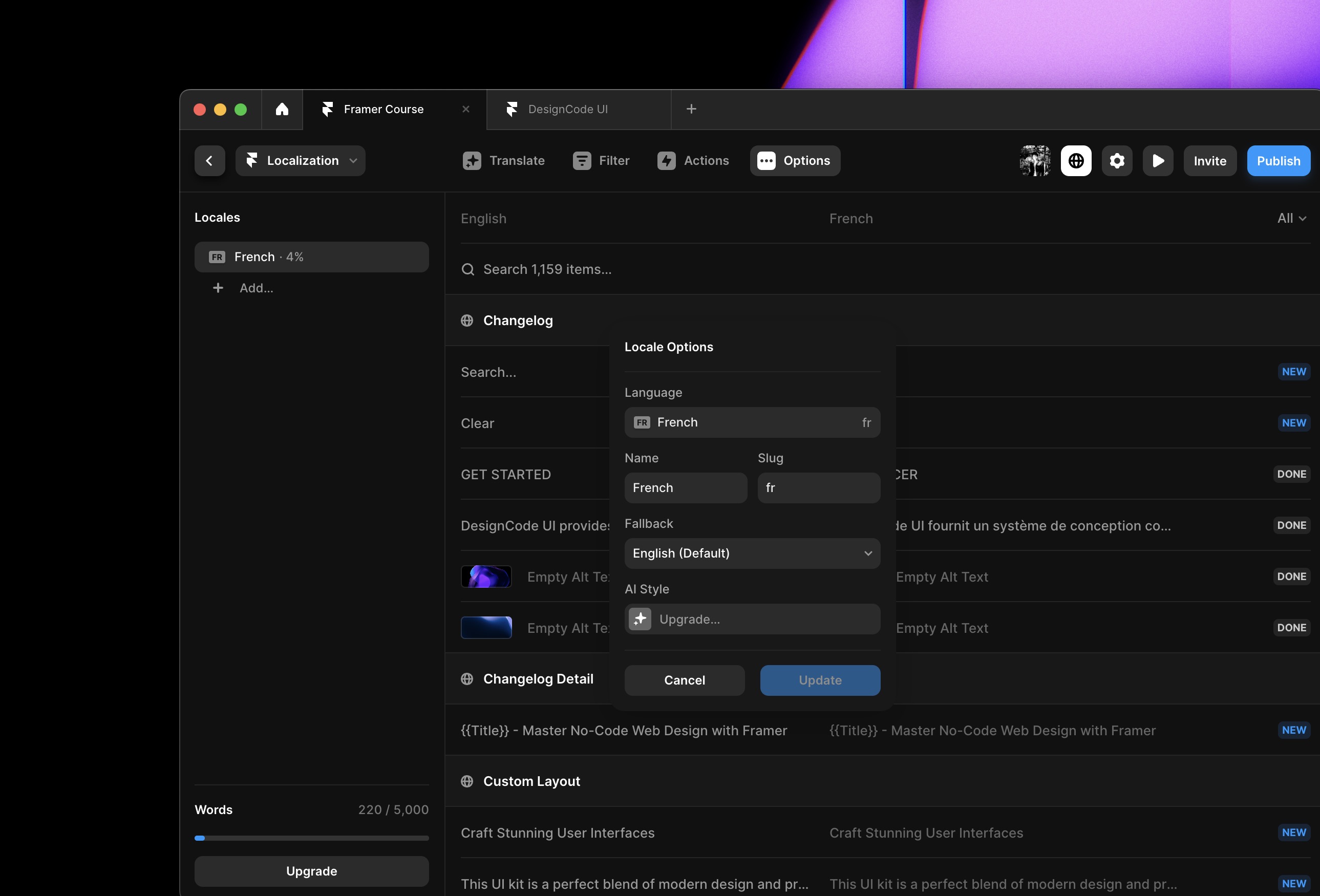A detailed screenshot of a software application is presented. The background of the interface is black with purple accents. The header features three circular buttons on the left, colored red, yellow, and green, reminiscent of typical window control buttons. Adjacent to these is a prominent white "Home" button.

The title "Framework Course" is displayed in bold white text against a black background. A secondary tab, labeled "Design Code.UI," is visible, but the primary focus is on the open tab highlighting a "Localization" section, evident from its placement in the upper left-hand corner.

Within this active tab, several submenu items are listed, including "Translate," "Filter," "Actions," and "Options," with "Options" currently selected and visibly highlighted. Additionally, several icons are aligned in a row: a user profile button, a world (globe) icon likely for language settings, a gear icon for settings, a play icon, an invite icon, and a conspicuous blue "Publish" button.

On the left panel, under "Locales," there is an indication that the French localization is 4% complete. This panel lists tabs for both English and French languages. The system is in the process of searching through 159 items while displaying a "changelog." A pop-up window titled "Locale Options" is focused on the French language settings, featuring a "Cancel" button and a blue "Update" button, confirming changes made to the locale-specific settings.